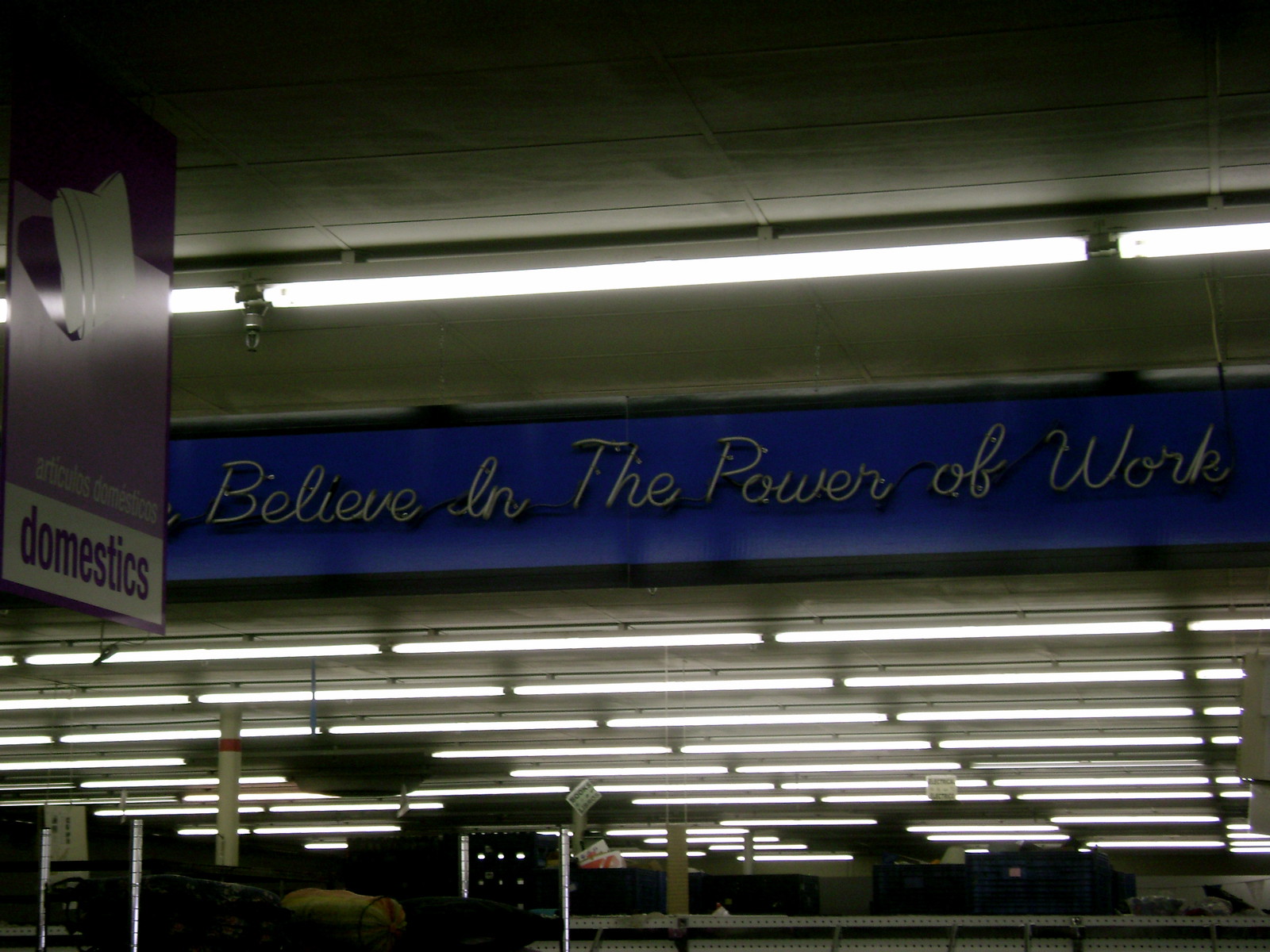This photo, likely taken inside a warehouse-style retail store, features rows upon rows of fluorescent lights that brightly illuminate the space, creating a well-lit but slightly shadowy atmosphere. In the foreground, the tops of white shelving units are visible, though the contents are a bit unclear, possibly suitcases or sleeping bags. A prominent blue neon sign in the center, though currently unlit, bears the cursive phrase "believe in the power of work," adding a somewhat Orwellian touch to the scene. In the upper left corner, a purple sign with the word "domestics" can be seen, along with a smaller text above it in Spanish, "Articulos Domesticos." This setup hints at the store's bilingual environment and its focus on work-related goods.